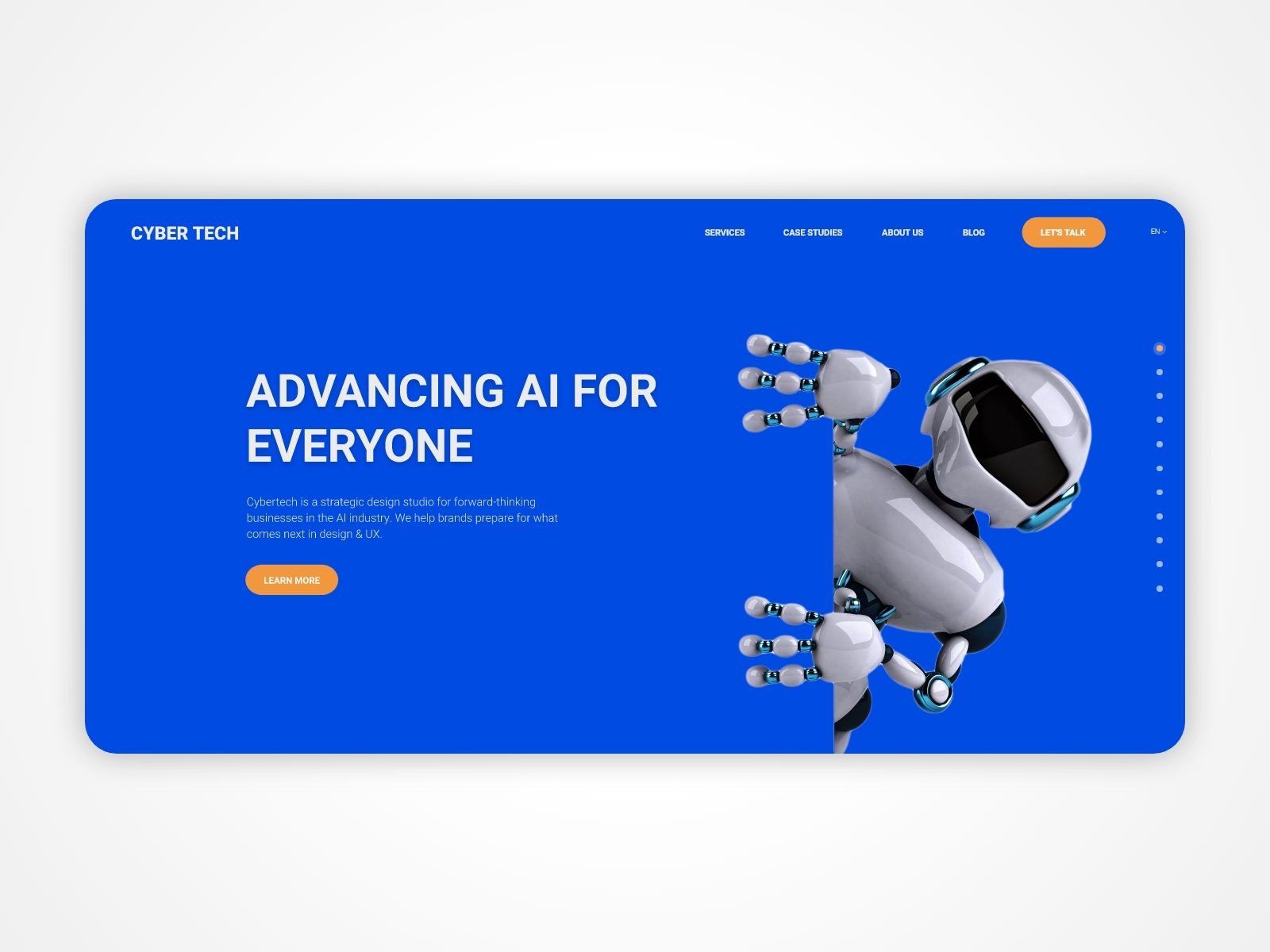**Detailed Caption:**

This image is a screenshot of a web page designed to emulate the shape of a cell phone's display, presented in a horizontal (landscape) orientation without the visible bezel or the phone itself. The overall background of the web page is gray, while the central, cell phone-shaped section of the screen is blue.

At the top left-hand corner of the blue screen, the word "CyberTech" is displayed in white text. To the right of this title, there are four clickable options, arranged horizontally, although their specific labels are not mentioned. Further towards the right, an orange button with white text reads "Let's Talk."

Prominently centered towards the left of the web page, there is a large text in white that boldly states "Advancing AI for Everyone," though there are additional words beneath this heading that are not legible. Directly below the unreadable text, there is another orange button labeled "Learn More."

On the right-hand side of the page, an illustrated robot is visible. The robot, characterized by a white body with a grayish-white sheen, is depicted holding a blue piece of paper in front of its chest and looking directly at the viewer. The robot's hands, which each have three fingers, are clearly gripping the paper. Visible joints at the robot's shoulders and elbows suggest articulations similar to human anatomy. The robot wears a helmet reminiscent of a motorcycle helmet, colored white with a dark visor, obscuring any facial features or eyes.